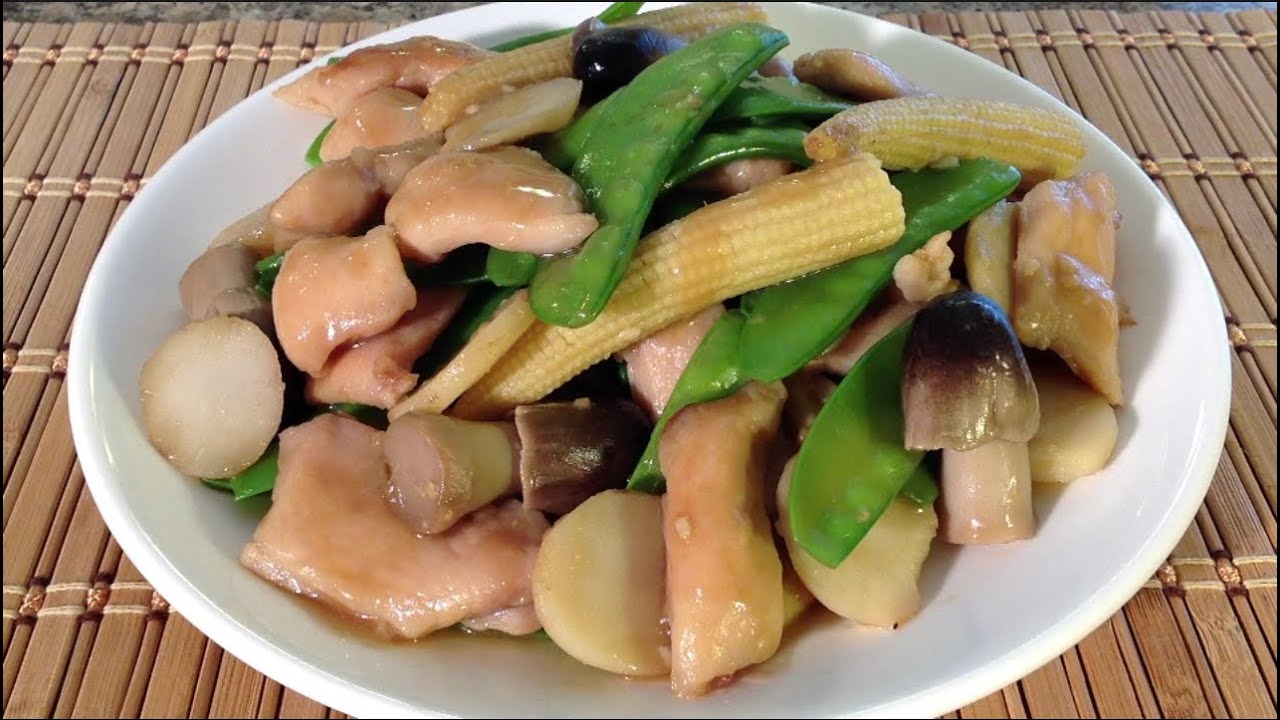The image showcases a white plate filled with a colorful and detailed Asian-style stir-fry. The dish includes an array of vegetables such as capped mushrooms, snow peas, baby corn, and ginger, possibly accompanied by Chinese potatoes. Adding to the mix are savory proteins, potentially chicken or pork, and a scattering of saltwater cashews. The ingredients are lightly coated in a brown sauce with a few sesame seeds speckled across the dish. This vibrant stir-fry sits on a honey-colored bamboo mat, composed of vertical wooden sticks connected by woven threads, which further enhances the Asian aesthetic of the presentation.